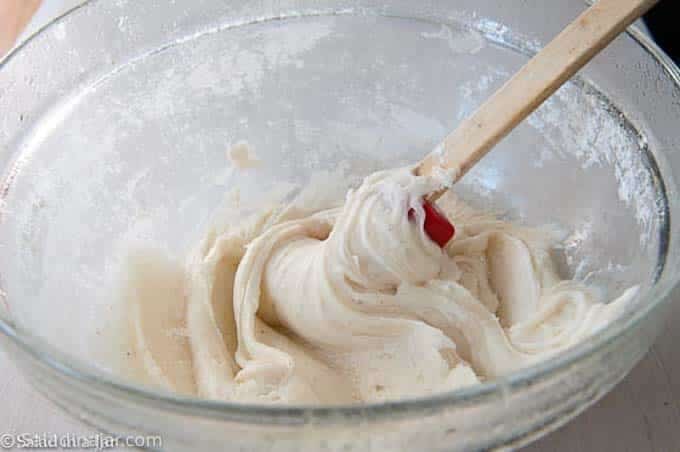The image depicts a clear glass bowl that dominates the frame, nearly filling the entire picture. Inside the bowl is an ivory-colored mixture that resembles either icing or a custard-like batter, being vigorously stirred. The mixture has a smooth, creamy consistency with white debris, possibly unmixed flour, clinging to the sides. The stirring is being done with a red-tipped wooden spatula. The bowl rests on a surface, but the background details are minimal due to the focus on the bowl. In the bottom left corner, a blurred website tag can be identified, showing an indistinct ".com" ending.